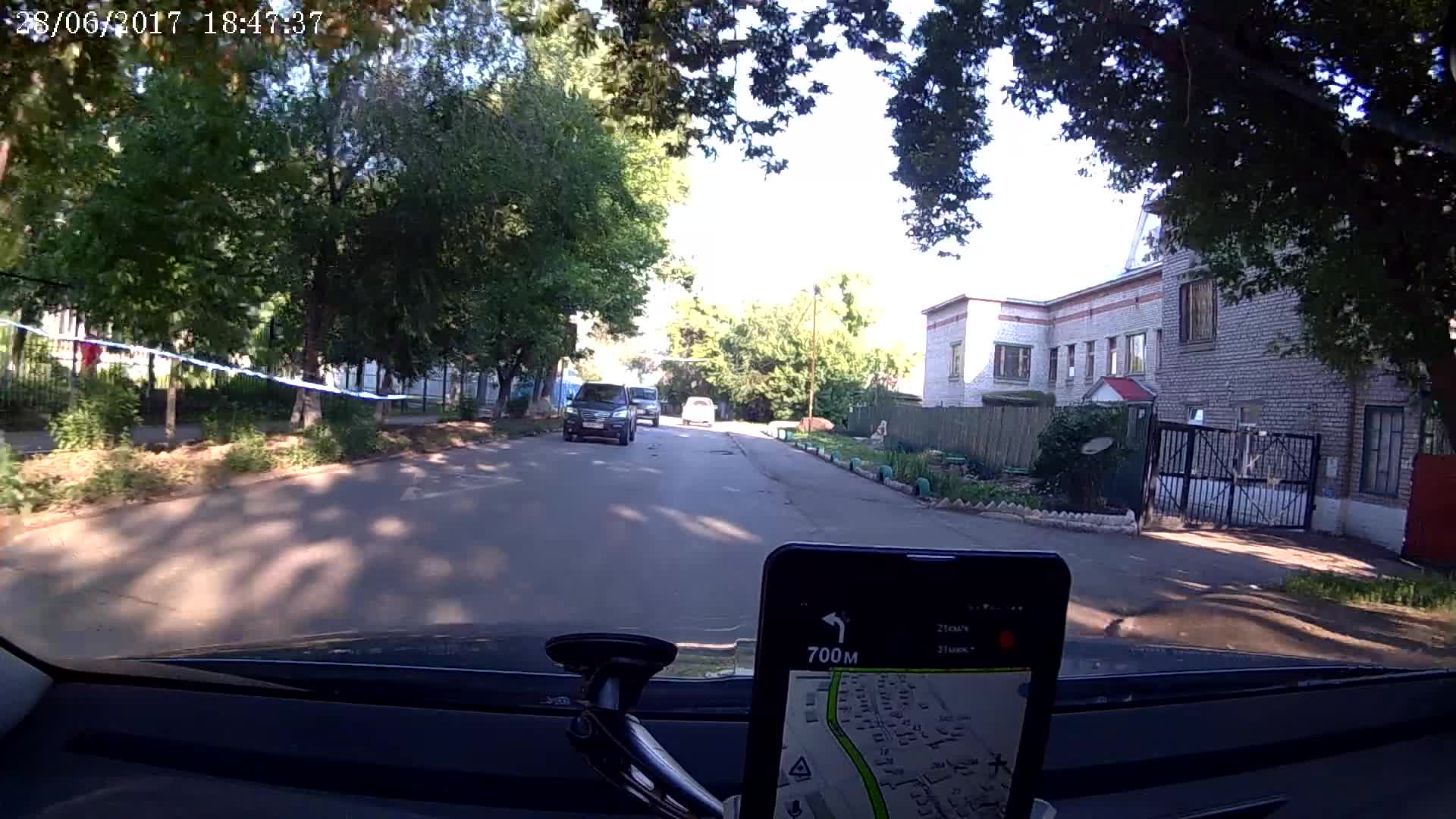The photograph appears to be taken from inside a car, looking out through a very clear front windshield. Attached to the windshield is a black mount holding a cell phone that displays a map, possibly indicating the use of a navigation app. Beyond the windshield, the scene depicts a sunny afternoon on a well-preserved residential street lined with overgrown trees that provide ample shade. The street includes a sidewalk with green shrubs and dirt, and a black fence on the left side. To the right, there is a gray brick building featuring numerous windows and a black gate with a diamond design. The road itself has a white triangle on the left side pointing towards oncoming traffic. Several vehicles are observed: two black cars approach the viewer, while a distant white truck travels in the same direction as the viewer. The date and time stamp "28-06-2017 18:47:37" in white text appears at the top left corner of the image.